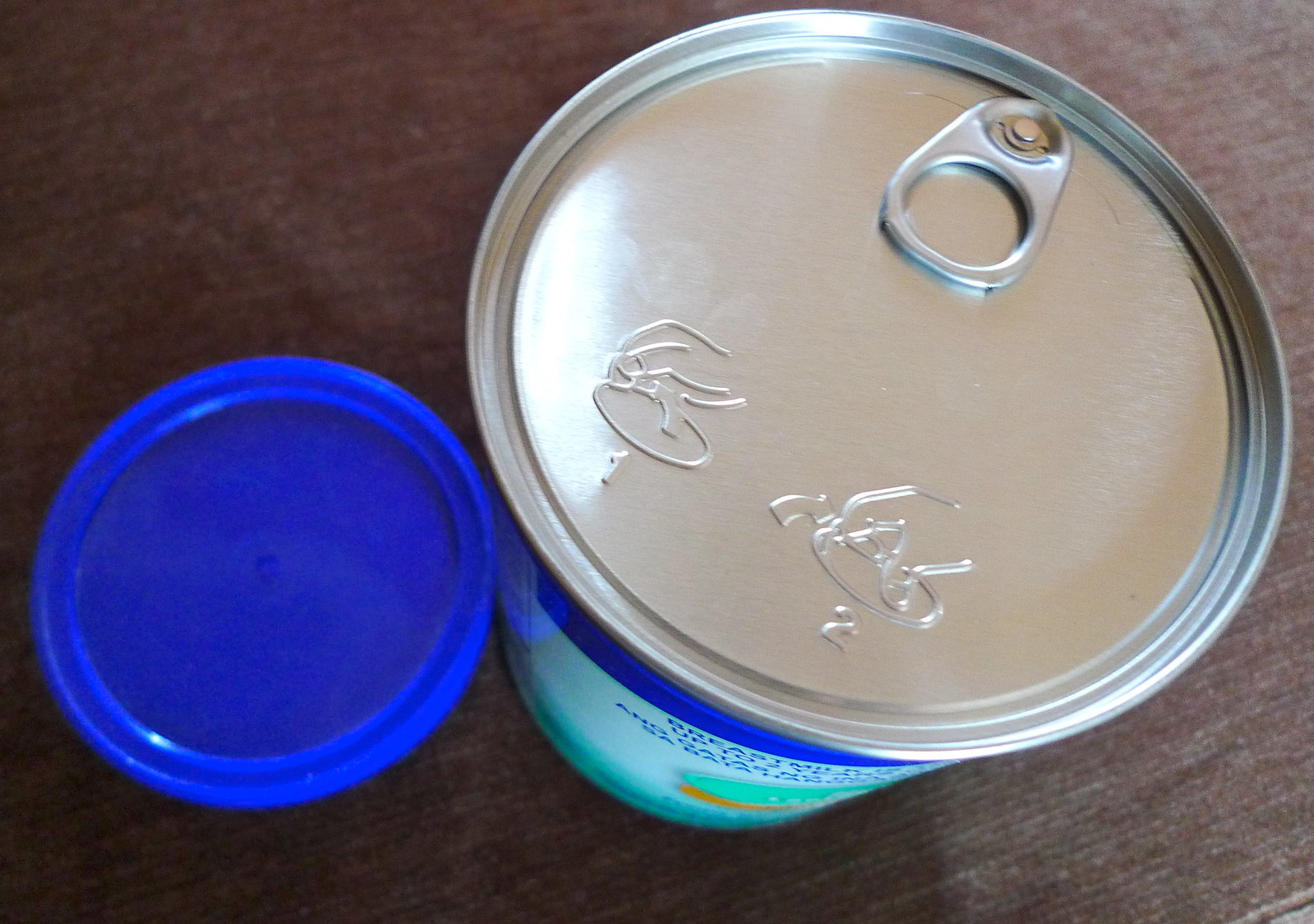A detailed photograph showcases the top of an enigmatic can, its contents unknown. The can itself is a soothing aqua color, with its aluminum lid removed and placed to the side. The lid features a two-step diagram that instructs how to lift and pull the tab, illustrated by a hand performing the action. A blue plastic cap, likely a part of the can, rests on a richly colored chocolate brown tabletop or countertop that exhibits a natural wood grain texture. Although partially obscured, part of the can's label is visible, displaying a design in yellow and a darker teal shade than the can's body. Some indistinct writing appears on the can, suggesting words like "mint bee" or "pretty," though they remain unclear. The image beautifully captures the curiosity and ambiguity of the can's contents.